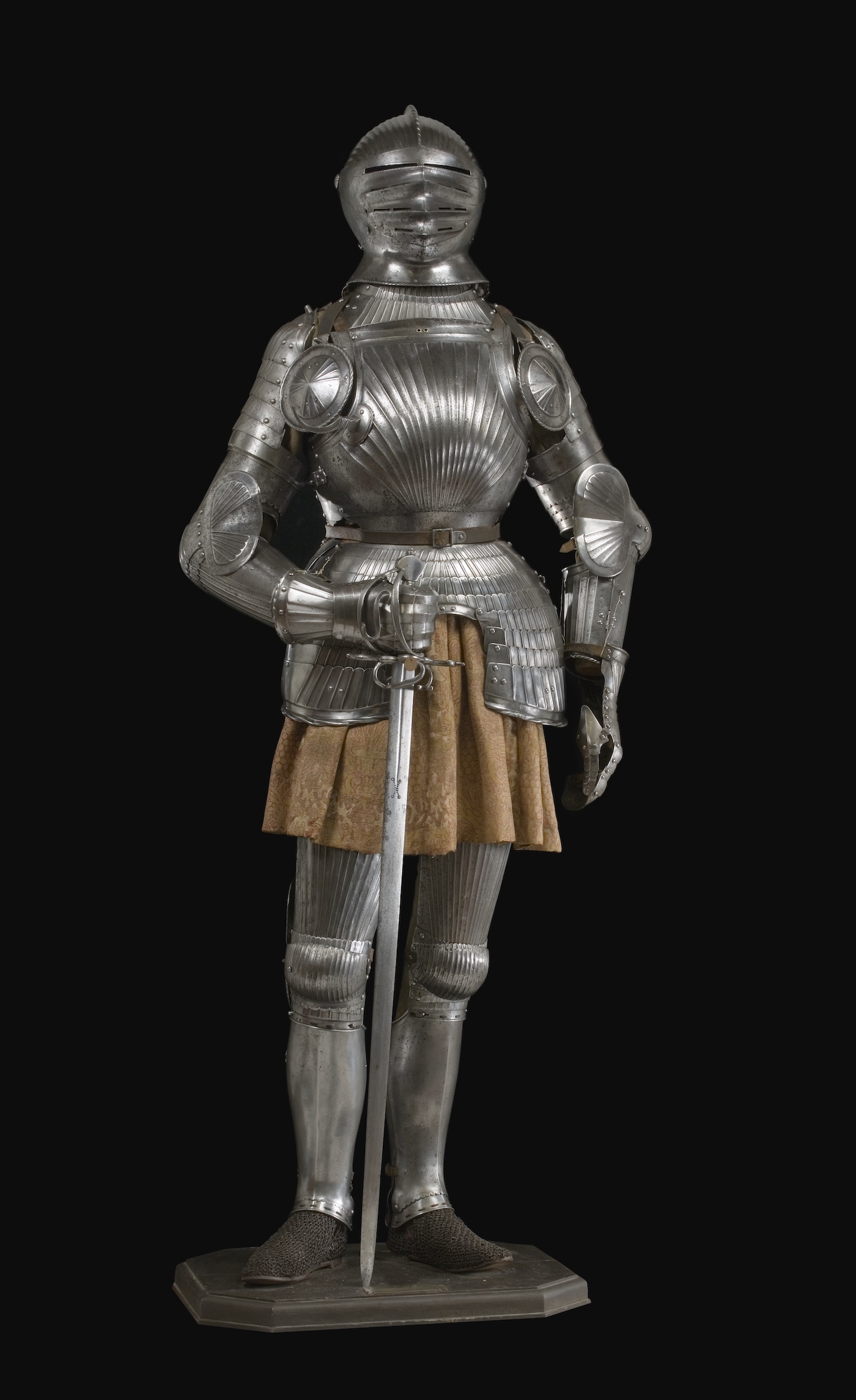The image depicts a solitary suit of knight's armor, strikingly positioned on a wooden geometric placard base against a plain black background. The silver armor, meticulously detailed, resembles a knight standing as if worn by an invisible figure. The helmet is fully enclosed with cutouts for the eyes and mouth, emphasizing the knight’s readiness for battle. The torso is clad in silver metal, complete with a belt at the waist, and below it, a light brown, burlap-like skirt extends to mid-thigh, adding a contrasting texture. The right arm is bent at the elbow, grasping a long, silver sword with its tip embedded firmly into the wooden base. Both arms and legs are encased in articulated silver plates, allowing flexibility at the elbows and knees. The knight's feet are covered with dark brown, chainmail-like shoes, adding to the historical authenticity. The photograph, devoid of any writing, people, or animals, focuses solely on the solitary, majestic figure of the armored knight, capturing a timeless image of medieval chivalry.